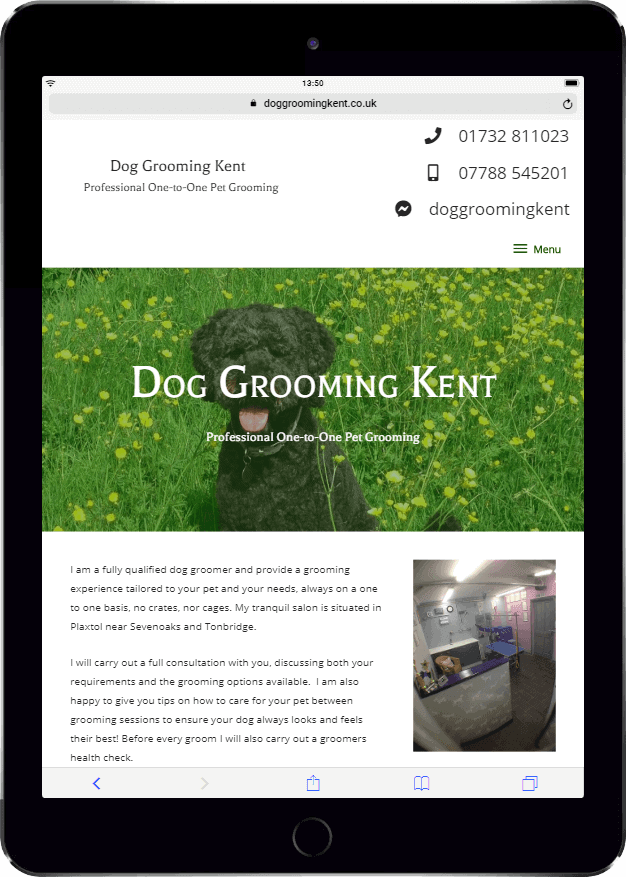The webpage for Doll Grooming Kent features a sleek design with key information prominently displayed. At the top of the page, the URL dollgroomingkent.co.uk is visible, and the current time is shown as 12:50 PM. Below this, there are contact details including a phone number, mobile number, and the Facebook Messenger handle "Doll Grooming Kent," allowing for easy communication.

On the left side of the page, a title reads "Doll Grooming Kent Professional 1-to-1 Pet Grooming" in bold letters. Beneath this title, there's an inviting image of vibrant yellow flowers against a lush green background. Adjacent to this is a charming picture of a black dog with its tongue playfully hanging out, overlaid with the same professional title in white letters.

The content further down the webpage describes the unique, personalized grooming experience offered by Doll Grooming Kent. The text reads, "I am a fully qualified dog groomer and provide a grooming experience tailored to your pet and your pet's needs always on a 1-to-1 basis. No crates nor cages. My tranquil salon is situated in Plaxtol near Sylvan Oaks Tonbridge. I will carry out a full consultation with you discussing both your requirements and the grooming options available. I am also happy to give you tips on how to care for your pet between grooming sessions to ensure your dog always looks and feels their best. Before every groom, I will also carry out a groomer's health check."

The visual and textual elements together create a welcoming and professional atmosphere, emphasizing the personalized and attentive care provided at Doll Grooming Kent.